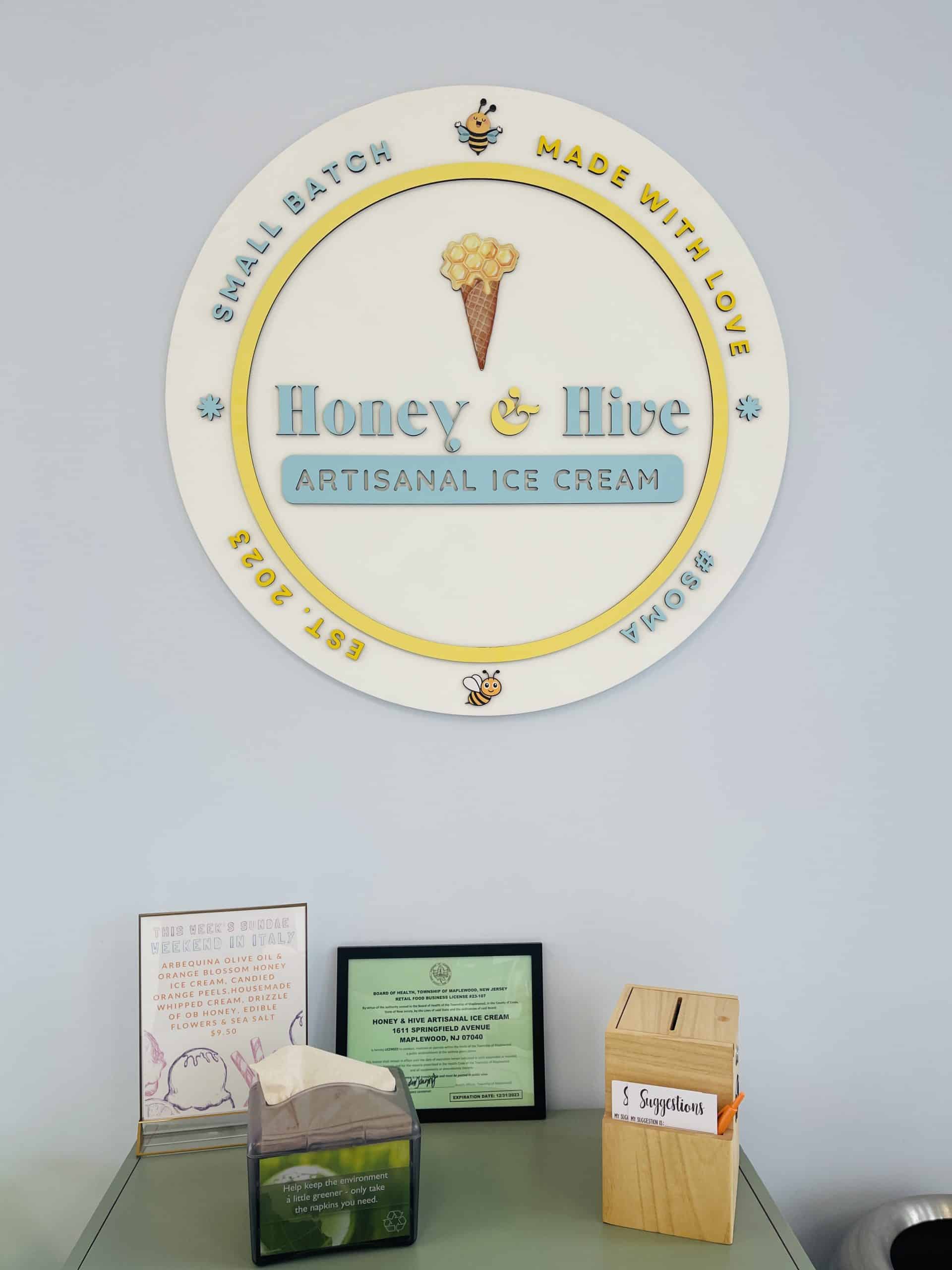The image captures a well-decorated office setting, showcasing the corporate logo of Honey and Hive Artisanal Ice Cream mounted on the upper half. The logo is circular, featuring light blue letters and illustrations. Central to the logo is an ice cream cone filled with honeycomb, surrounded by charming bees. In delicate yellow letters, the logo proudly displays the messages: "Small Batch," "Made with Love," "Established 2023," and "#SOMA." Below this visually appealing sign, which is set against a white backdrop, a desk painted green holds various items including a certification, tissue box, wooden box, and a napkin dispenser. Additionally, the desk provides the company's address, 1611 Springfield Avenue, Maplewood, NJ, and details this week’s special sundae called "Weekend in Italy." This sundae features Arbequina Olive Oil & Orange Blossom Honey Ice Cream, Candied Orange Peels, Housemade Whipped Cream, Drizzle of Honey, Edible Flowers, and Sea Salt, priced at $9.50.